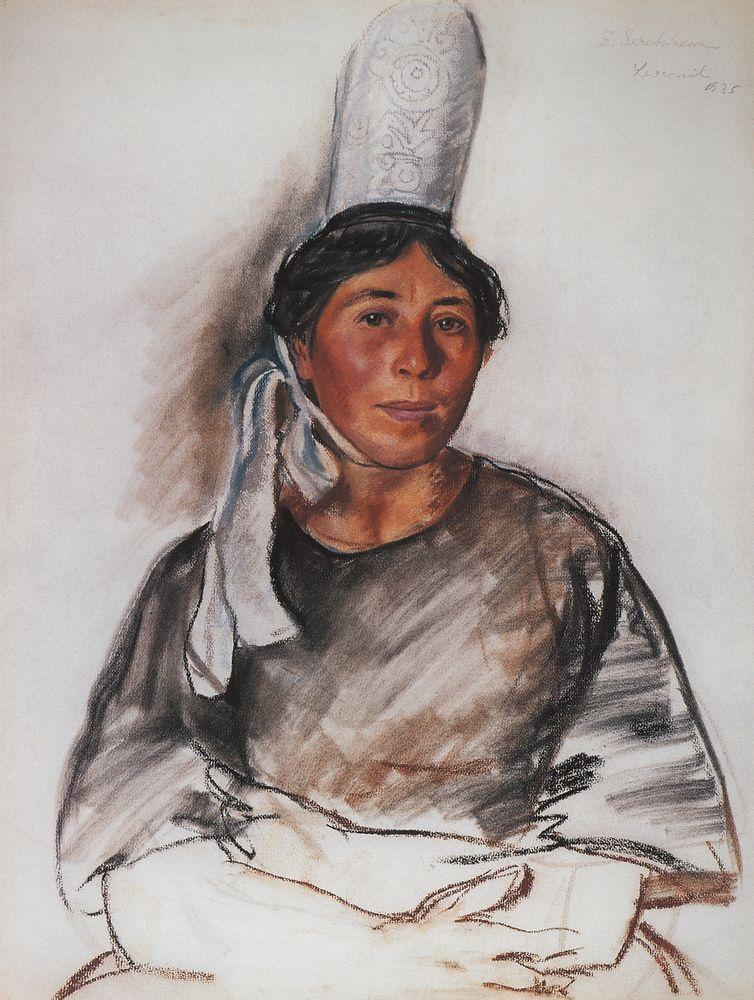This detailed pastel sketch, titled "Young Breton" by Zinaida Serebryakova, created in 1934, portrays a woman of dark complexion and possible Native American or South American descent. The woman appears to be in her early 30s with short black hair, adorned with a white bow that ties to the left side of her face. She wears a black and brown shaded tunic, with her arms folded across her chest and an expressionless face gazing directly at the viewer. Atop her head rests a tall cylindrical white hat, resembling the Pope's mitre, decorated with intricate light gray designs and secured by a ribbon around her neck. The background is predominantly a light beige wall, with black and brown outlines sketching the setting around her. The artwork exhibits an expressionist style, with certain areas meticulously detailed while other parts remain simply sketched, focusing the viewer’s attention on the central figure.